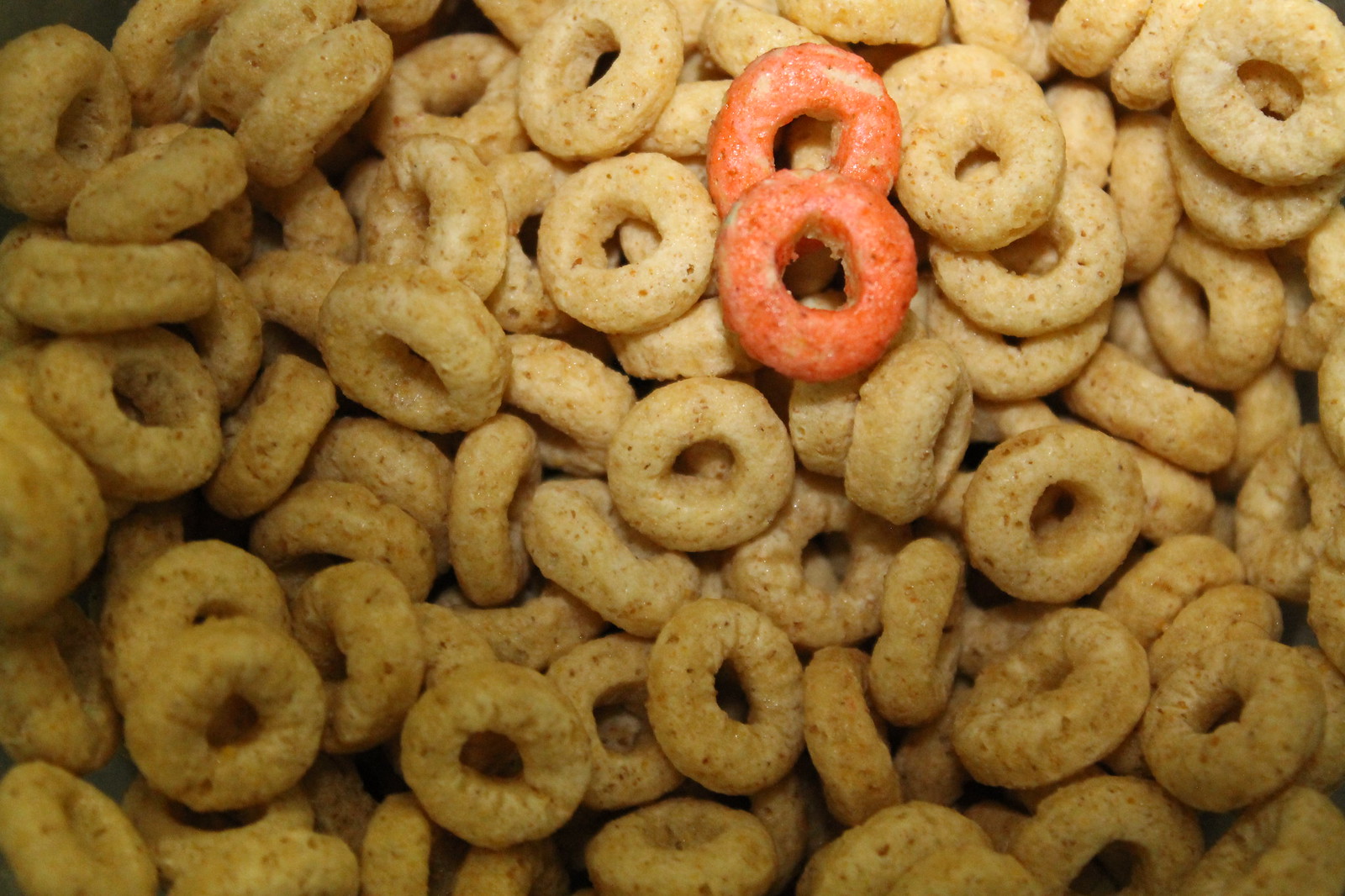This image is an up-close photo of a multitude of light tan, round-shaped Cheerios, complete with distinctive donut-like holes. Among these uniformly colored cereal pieces, there are two unique salmon pink loops, situated in the upper middle center of the picture, stacked together to form a figure-eight shape. The pink cereal pieces, possibly flavored, stand out prominently against the otherwise homogenous backdrop of Cheerios. The regular Cheerios are tan with darker brown speckles, adding to their texture. The lighting in the photo is uneven, with noticeable shadows occupying the bottom part, far left, and the bottom right corner, contrasting with the bright light illuminating the top and the top right areas. The striking colors and lighting nuances draw attention to the focal point – the two pink loops amid the sea of tan Cheerios.